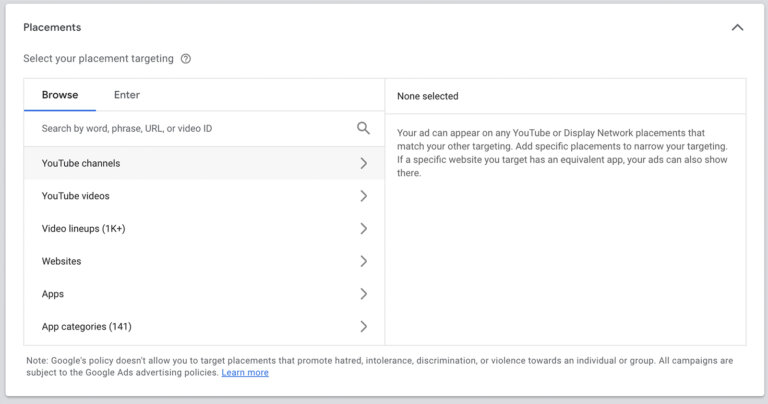Screenshot Detailing Placement Targeting Options for YouTube and Display Network Ads

The image is a slightly blurry screenshot displaying a user interface for selecting ad placement targets, featuring a white background with black text. 

At the top, the heading reads "Placements" with a prompt underneath: "Select your placement targeting." Beside this text is an icon of a circle with a question mark inside, likely for help or more information.

Below the heading, there are two options in blue underlined text labeled "Browse" and adjacent to it, the word "Enter" which is not underlined. Following this, a prompt suggests users "Search by word, phrase, URL, or video ID."

Further down, expandable options are listed, each with a right-facing arrow indicating they can be opened to reveal more details:
- "YouTube channels"
- "YouTube videos"
- "Video lineups (1K+)"
- "Websites"
- "Apps"
- "App categories"

To the side, there is a box indicating "None selected," which likely populates with selected placements.

At the bottom, a note specifies: "Your ad can appear on any YouTube or Display Network placements that match your other targeting. Add specific placements to narrow your targeting. If a specific website you target has an equivalent app, your ads can also show there."

Additionally, a highlighted caution states: "Note: Google's policy does not allow you to target placements that promote hatred, intolerance, discrimination, and so on."

This screenshot appears to be from an ad management platform, providing a comprehensive set of options for advertisers to refine where their ads will be shown across YouTube and the Display Network.